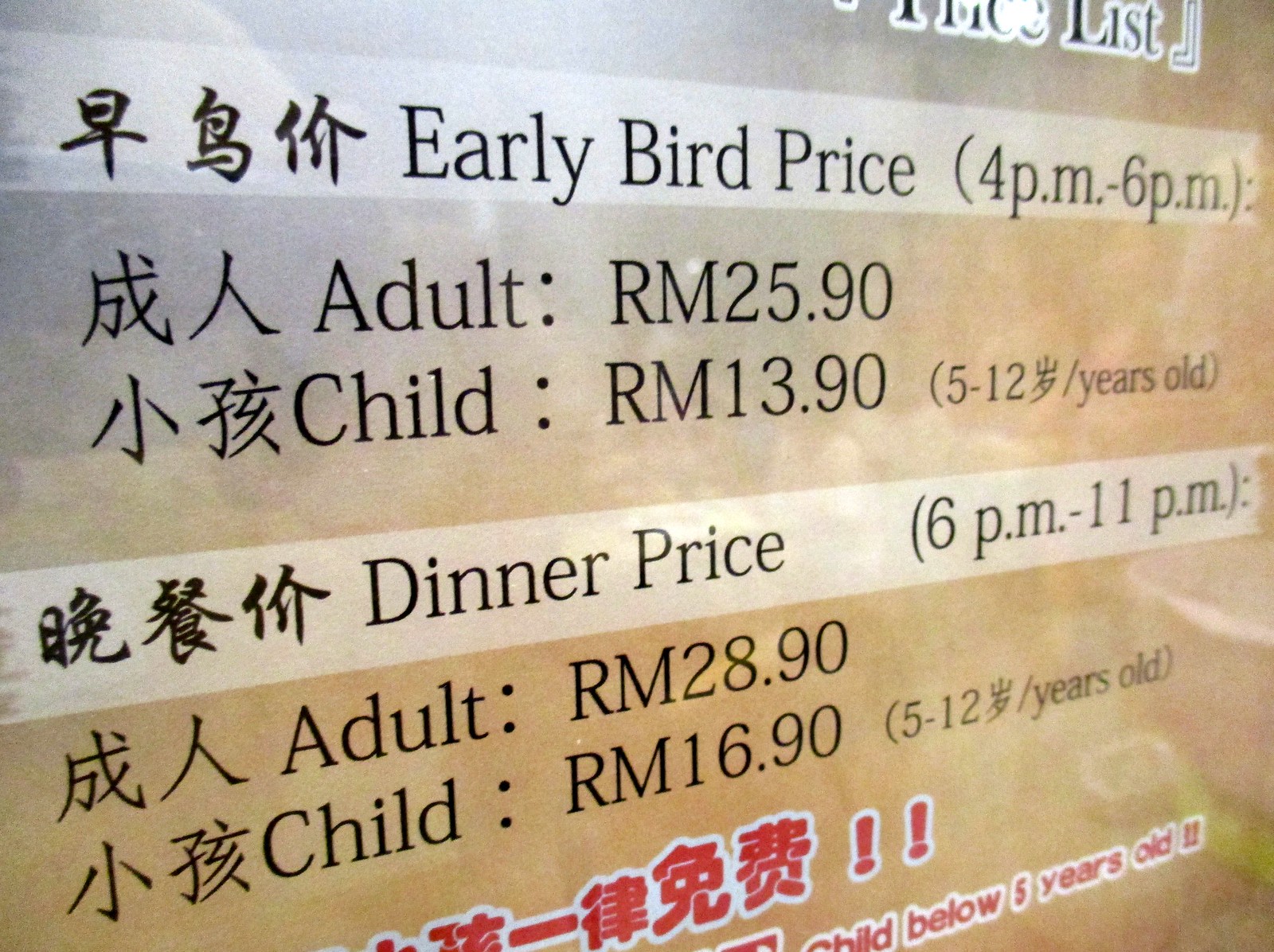This horizontal rectangular image is a close-up photograph of a menu posted on a wall, viewed at an angle, making the left side appear larger and closer than the right. The background primarily features a reflective brown color with lighter tan horizontal stripes in the upper-right corner, adding a bit of glare. At the top of the menu, though partially cut off, there is some text in Oriental characters above a lighter white line that prominently reads "early bird price" in black print with "4 p.m. to 6 p.m." in parentheses next to it. Below this line, on the brown background, the menu lists prices for adults and children, specifying that "adult rm25.90" and "child rm13.90 (5-12 years old)" are the early bird prices.

A light tan banner below these prices displays more Asian characters, followed by "dinner price (6 p.m. to 11 p.m.)" in black print. Underneath this section, against the brown background again, are the dinner prices: "adult rm28.90" and "child rm16.90 (5-12 years old)." Further down, there are red Oriental characters outlined in white, accompanied by two exclamation points. At the bottom of the image, partially visible text reads "child below five years old" with two exclamation marks. The detailed menu combines both Oriental characters and English, providing clear information on pricing for different times and age groups.